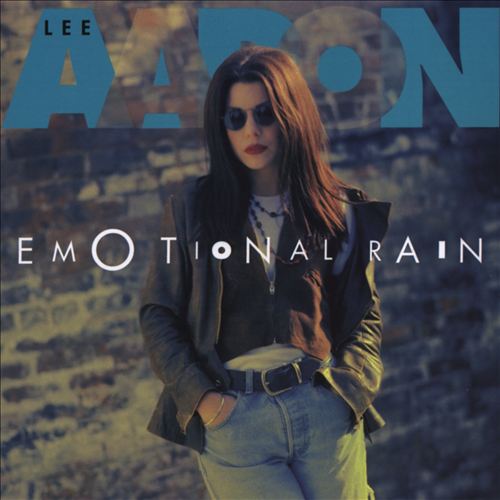This image appears to be an album cover featuring a woman posing against a brick wall as the central figure. Her outfit consists of jeans paired with a dark brown cropped hoodie layered under a black leather jacket with a zipper and long sleeves. She accessorizes with a black belt, a large blue-beaded necklace, a gold bracelet, dark red lipstick, and circular sunglasses, highlighting her long brown hair parted in the middle. The text "Lee Aaron" is displayed at the top of the cover, with "Lee" positioned on the top left and "Aaron" across the top, where the letters A-A-R-O-N alternate between blue and transparent, blending somewhat into the backdrop. In the middle of the image, white text spells out "emotional rain" with distinctively sized letters that create a unique visual effect. Notably, the 'O' in 'emotional' is a circle, and the 'I' in 'rain' is a solid block, adding to the artistic design.